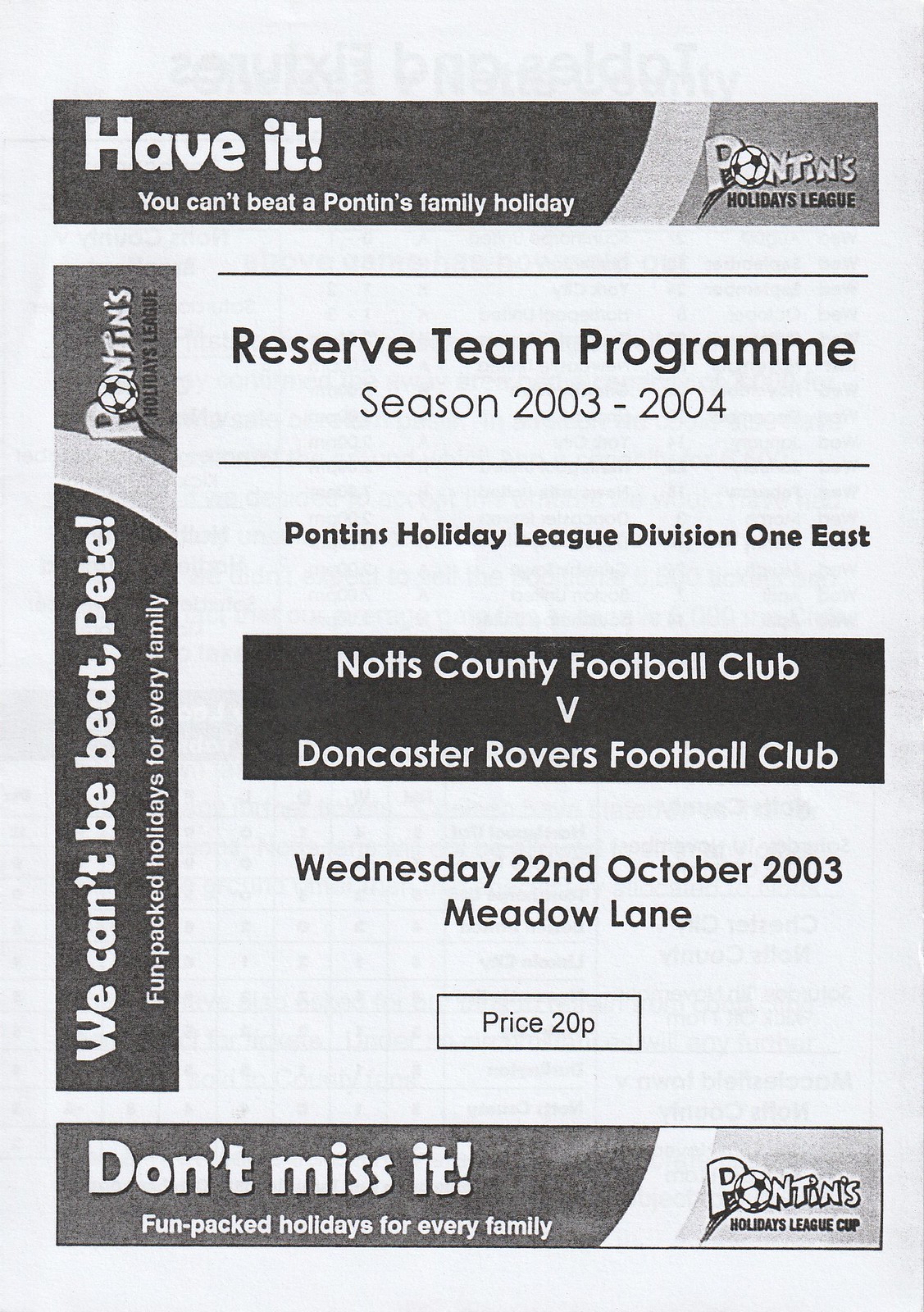This is a black-and-white flyer for a soccer game featuring detailed text and graphics. At the top, a horizontal banner reads: "Habit, you can't beat a Pontins family holiday." A similar banner on the left side says: "We can't be beat! Fun-packed holidays for every family." At the bottom, another banner reiterates: "Don't miss it, fun-packed holidays for every family," and includes the Pontins logo. Additionally, the flyer features a logo with a soccer ball and the text "Pontins Holiday League." The main body of the flyer announces: "Reserve Team Program, Season 2003-2004, Pontins Holiday League, Division 1 East: Knott's County Football Club vs. Doncaster Rovers Football Club on Wednesday, 22nd October 2003 at Meadow Lane." The ticket price is stated as £20.